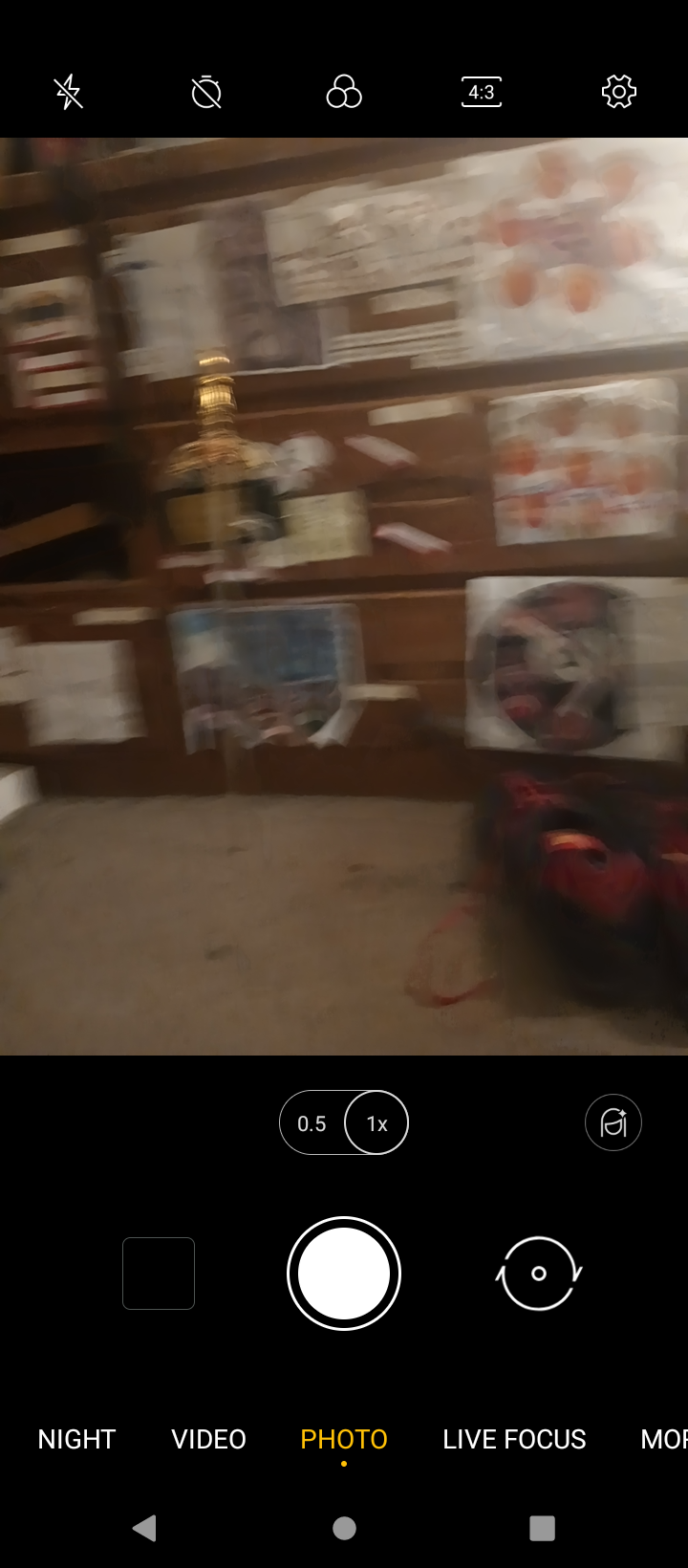The image is a screenshot taken from a cell phone. At the very top, a horizontal black rectangle displays standard white cell phone symbols. Below this is a tall square photograph, although quite blurry, showing some papers with drawings or diagrams affixed to a brown wall. The floor beneath the wall is concrete. Towards the right edge of the photograph, there is a black square with red markings. At the bottom, the screen has a black background with a white circle in the middle, indicating the shutter button used to take photos on a cell phone. Below the shutter button is a strip of writing: 'video' in white to the left, 'photo' in orange in the center, and 'live focus' in white to the right.